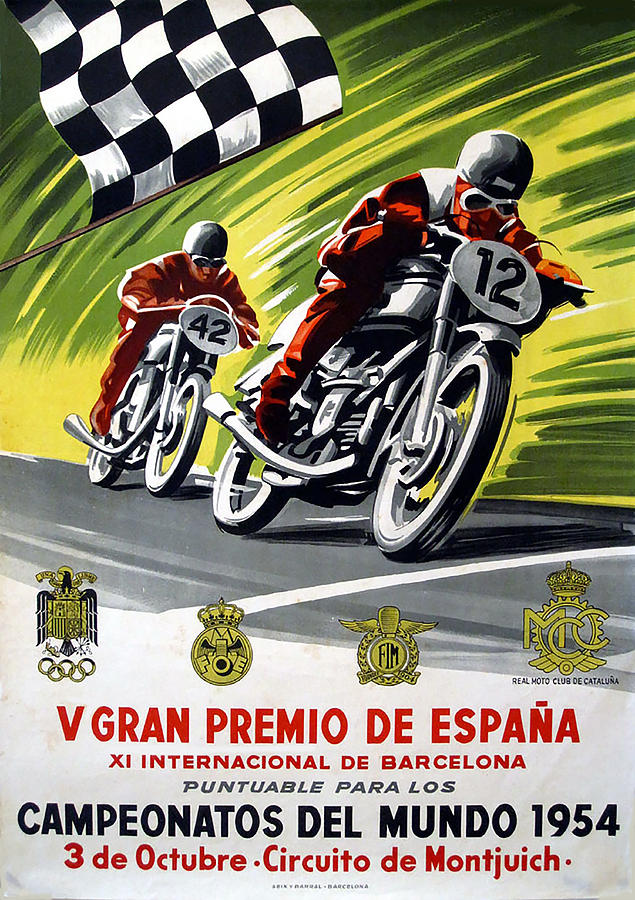This vibrant vertically-aligned poster from 1954, presumably in Spanish, showcases a dynamic scene of an international motorcycle race held in Barcelona. Dominating the top portion are two motorcycle racers clad in striking red suits, black helmets, and goggles. The foreground features the number 12 racer, while immediately behind, another racer on a similar bike is marked with the number 42. Both motorcycles are mainly black, white, and gray. They appear to be racing at high speed, illustrated by energetic streaks of green and yellow in the background.

A checkered flag, signifying the race's finish, is prominently displayed at the top left, attached to a flagpole. The middle section of the poster is adorned with four gold emblems, including one stating "FIM" and another labeled "Real Moto Club de Catalina." 

Text in bold red and black includes the event title, "V Gran Premio de España," alongside "XI Internacional de Barcelona," and highlights that this grand event took place on October 3, 1954, at the Circuito de Montjuic. The text also notes, “Puntable para los Campeonatos del Mundo,” indicating that the competition was part of the World Championship series.